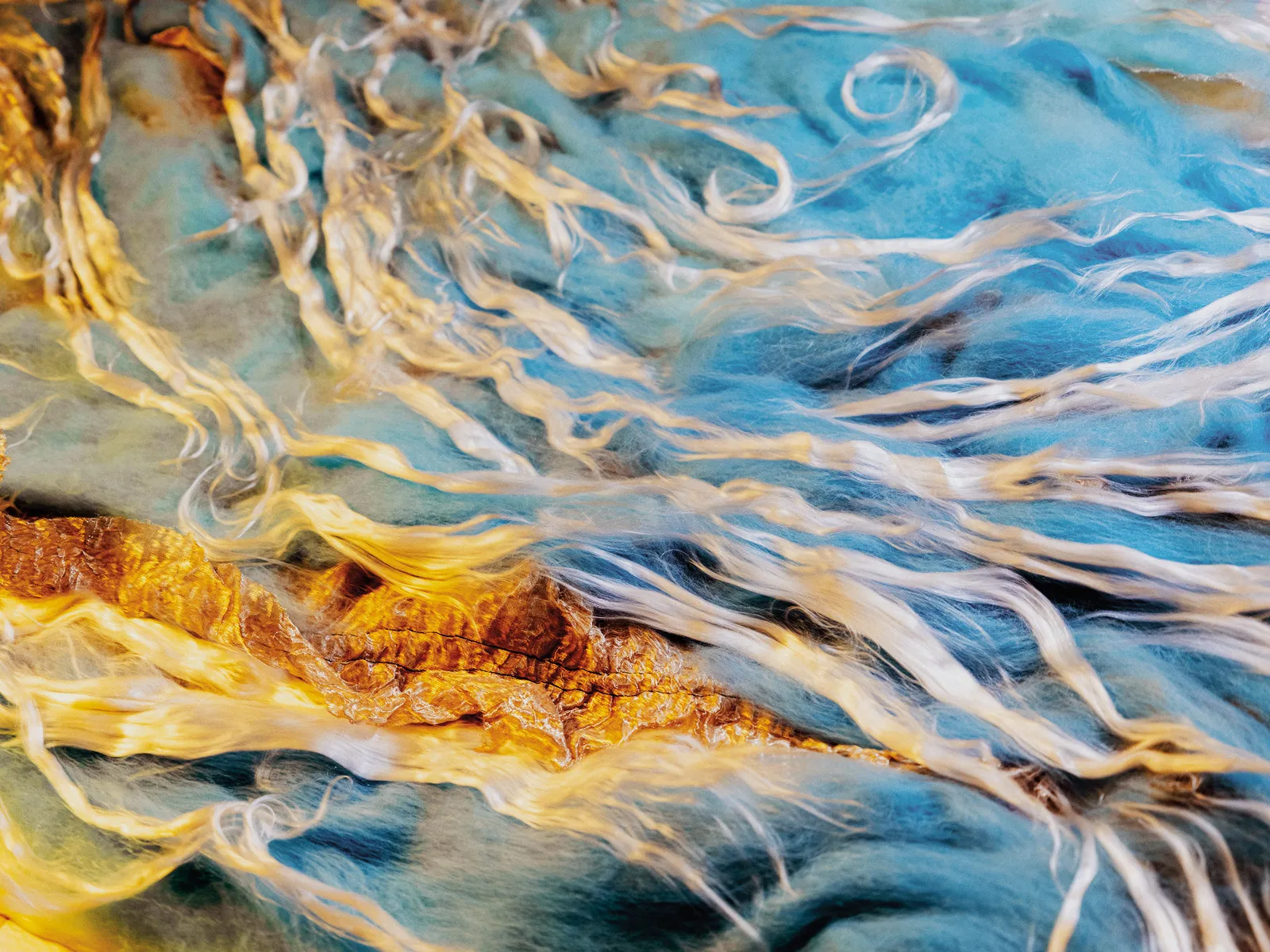The artwork captures an abstract outdoor scene featuring a strikingly vibrant and surreal landscape. Streams of white, filament-like bands meander through a vast, blue sky, evoking a sense of ethereal movement. Dominating the foreground is a group of imposing, orange and golden rocks, arranged in a triangular fashion, reminiscent of a mountain range or rocky spit extending from the middle left edge of the image downward to the right at a slight angle. Amidst the rocks, there's a natural arch formation that seamlessly blends with the terrain. The white bands crisscross the scene diagonally from the bottom right toward the top left, adding dynamic tension to the serene tableau. The overall composition is fluid, with the white filaments and soft, blue expanse seemingly in perpetual motion, suggesting both the tranquility and the relentless energy of nature.